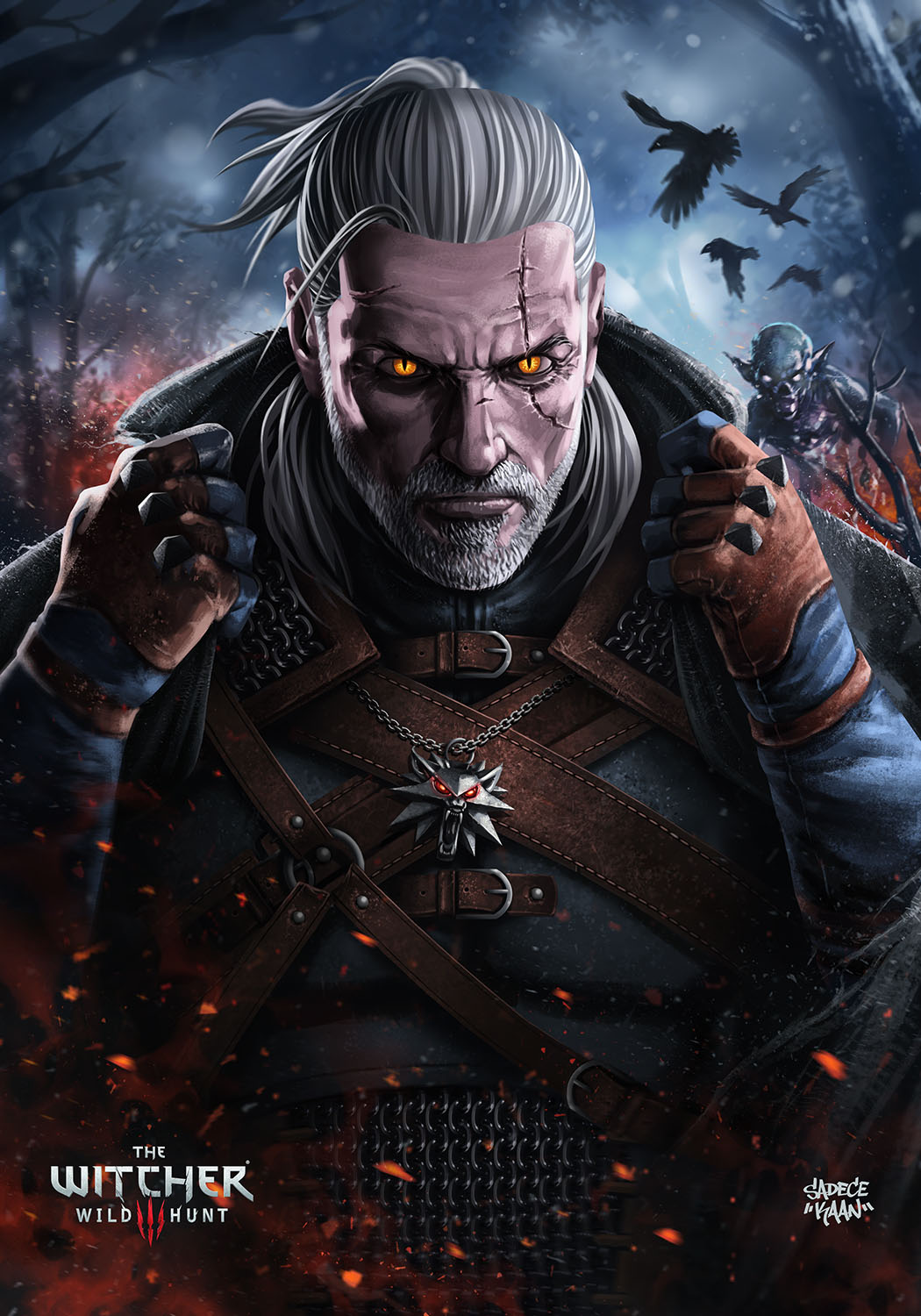The image appears to be a cover of a fantasy video game titled "The Witcher: Wild Hunt," indicated by silver letters at the bottom left corner of the image, with a red pitchfork-like symbol between "Wild" and "Hunt." The setting is dark and foreboding, featuring a grayish, snowy sky with dark-colored crows or ravens flying in the top right corner and barren trees to the left. In the foreground, a male character with distinctive features stands prominently. He has stringy, gray hair pulled back into a ponytail, intense glowing yellow cat-like eyes, and a deep scar running from his forehead through his left eye down to his cheek. His skin is light gray, and he sports a trimmed white beard and mustache.

He is wearing dark blue and brown battle armor adorned with numerous leather belts. His gloves are a matching color, with brown around the knuckle area. Hanging from his neck is a medallion resembling a wolf with red glowing eyes and fangs. The character appears vigilant, with his hands gripping the collar of his armor. In the background to his right, there is a menacing, zombie-like creature with glowing eyes peering over his shoulder. The overall atmosphere is eerie, reinforcing the dark fantasy theme of the game.